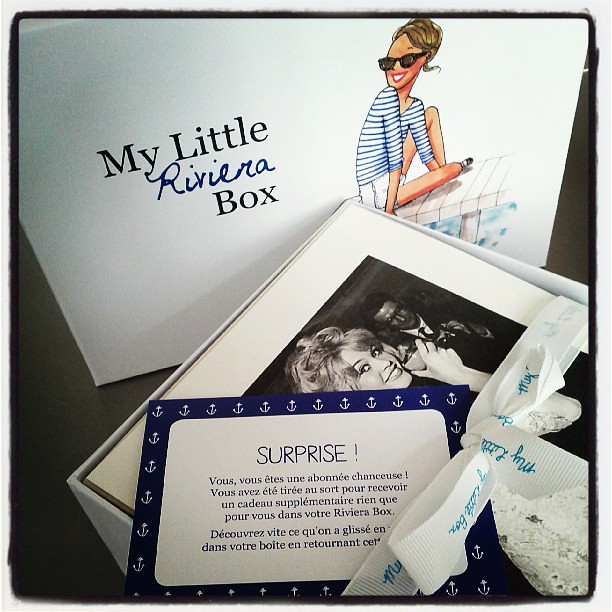This square image depicts a slightly opened gift box, tilted diagonally with its top cover standing upright at the back. The box’s white cover features a drawing on the right side of a blonde woman with a blue and white striped shirt, white shorts, and dark sunglasses, sitting on a white wooden dock over a body of water. Above the drawing, the text reads "My Little Riviera Box" in black letters. 

The bottom part of the box, oriented to the bottom right of the image, reveals its open interior. Inside, there is a white-framed photograph of a poised woman with a fancy hairstyle and a man in the background. The photograph has a bow with blue script wrapped around it. The setting and style of the image suggest it is a depiction of a thoughtfully curated gift box containing special surprises.